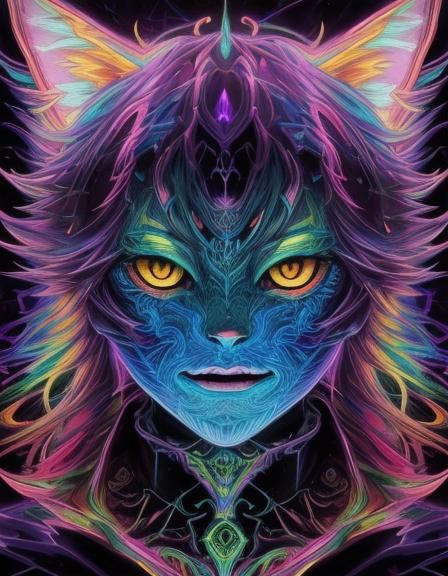This piece is a striking digital artwork featuring a stylized neon-colored Catwoman. The figure is adorned with vivid and contrasting hues, showcasing her otherworldly beauty. Her skin is a neon bluish color with swirly patterns, and her face is accentuated by bright, slanted eyes in shades of yellow and orange with dark pupils. Her lips are painted a thin purple, while the outer parts of her face transition to a striking purple hue, complemented by a light green forehead.

Her long, flowing hair cascades down with a mesmerizing mix of purples, accented with highlights of green, blue, yellow, red, and pink, enveloping her head and neck. Protruding cat-like ears, light-colored in shades of pink, light green, and light orange, add to her feline allure. She dons a distinctive green necklace featuring a teardrop element, resembling a stylized peacock feather, and a prominent green diamond at her neck. Diamond-shaped gems of varying purples and blues adorn her forehead, enhancing her mystical appearance.

This captivating artwork melds human and feline traits into a luminous, neon figure, with each detail emphasizing her ethereal and fantastical presence.